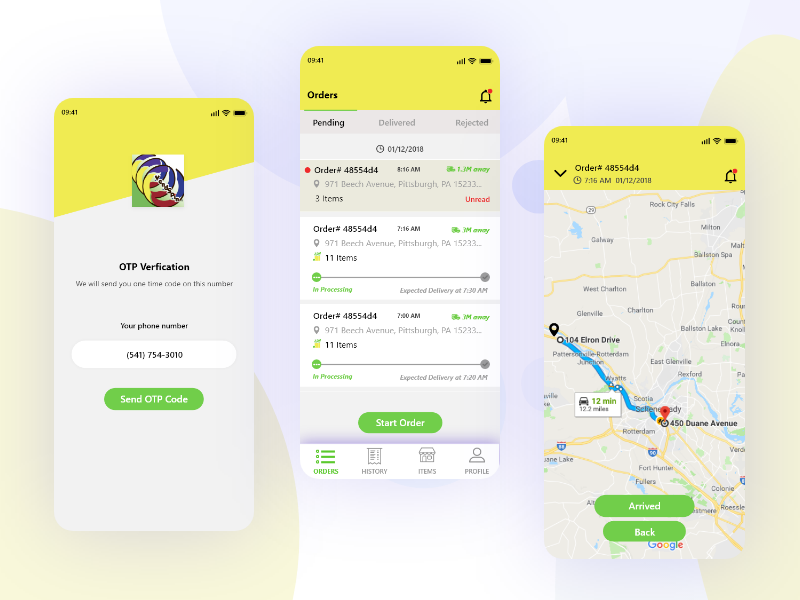The image displays the screens of three smartphones. In the top left corner of each screen, the status bar indicates the time as 9:41, with full cellular bars, a strong Wi-Fi connection, and a fully charged battery. The top of the first screen displays a glimpse of something yellow.

On the screen, there is a square graphic comprised of blue, yellow, and red sections. Below this, there is a text box for OTP verification with a message saying, "We'll send you one token on this number. Your phone number is 541-754-3010." Below this, a green rectangular button reads "Send OTP code."

The center screen appears to show an order management interface with sections labeled "Pending," "Delivered," and "Rejected." This section details order information such as an order number "48554D4" and a timestamp "8:16 AM." The delivery address is listed as "8971 Beach Avenue, Pittsburgh, Pennsylvania," with three items included in the order. Another timestamp of "2:16 AM" is visible, alongside information of 11 items in an order.

The bottom of the screens display navigation options: "Orders," "History," "Items," and "Profile."

Finally, the third screen shows additional order details for "Order number 48554D4," with timestamps "7:16 AM" and a date "06-12-2018." It also includes a blueprint route from "104 Alan Drive to 458 Duane Avenue," with a green label marked "Arrived" and a back button.